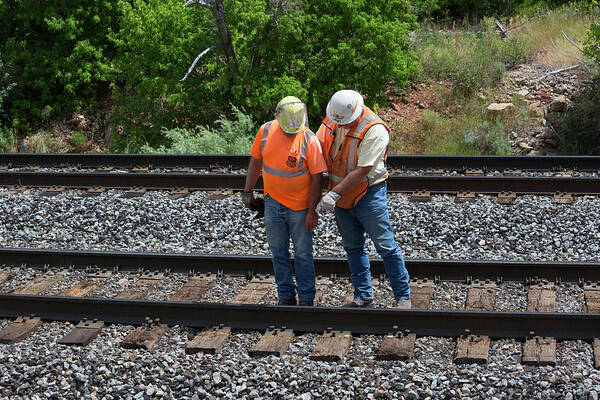In this outdoor photo taken during the day, two men, possibly engineers, are seen working by railroad tracks. Both men are dressed in blue jeans and hard hats—one wearing a bright orange safety vest over a yellow short-sleeve shirt and the other in an orange t-shirt with reflective stripes around the midsection and shoulders. The man in the orange vest is pointing at the track, while the other, who is standing to his left, appears to be looking down at it. Both men are also wearing boots, though the metal rail partially obscures their feet. They are positioned on the track closest to the viewer, with a parallel set of tracks right behind them. The ground is covered in rock and gravel, and the background features lush green trees and plants, suggesting a summer or late spring setting.